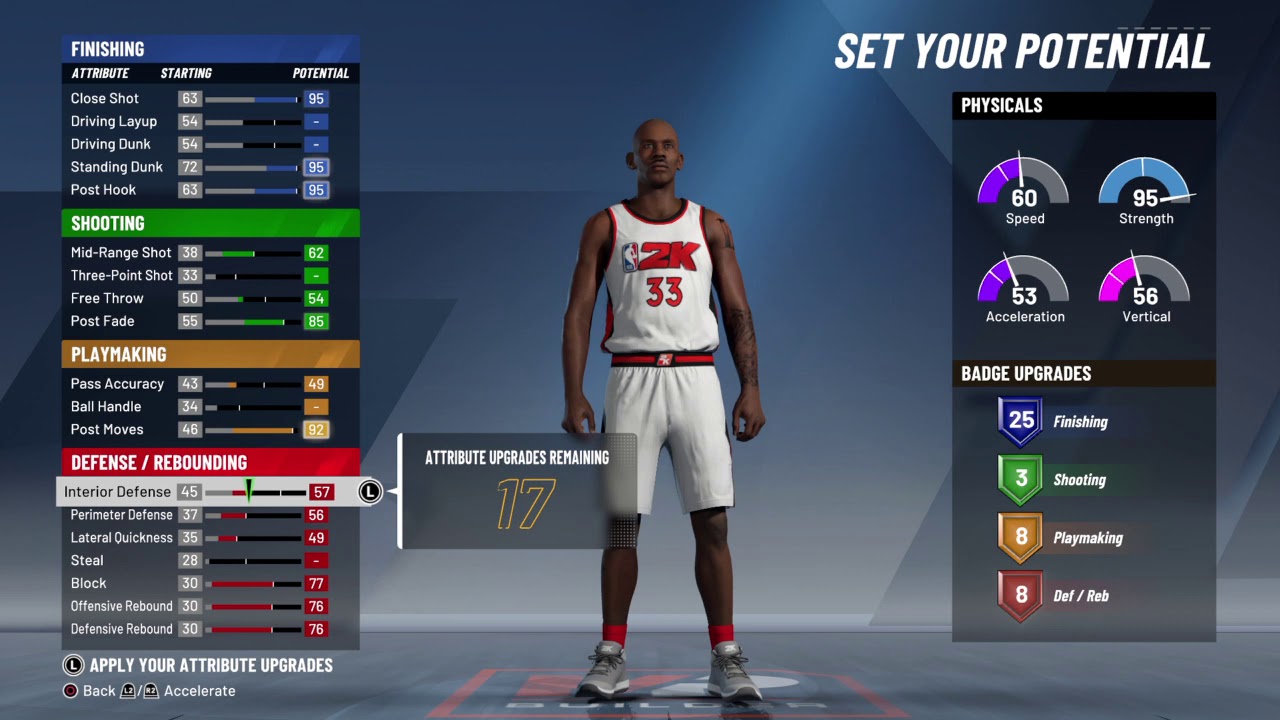This screenshot is from a basketball video game's settings and customization section, where players design and enhance their characters. The focus of the image is a character customization screen, featuring a player standing in a studio setting with a professional backdrop. The character, a black man resembling Michael Jordan, is dressed in a distinctive white basketball uniform. This uniform includes an NFL white jersey and pants, adorned with the NBA logo on the right chest along with a red number 33 and the "2K" branding.

On the right-hand side of the screen, there is a panel titled "Set Your Potential," displaying four gauges that represent different attributes: speed, strength, acceleration, and vertical. The current values shown are 60 for speed, 95 for strength, 53 for acceleration, and 58 for vertical, indicating the player's potential in these areas based on the positions of the gauge meters.

On the left-hand side of the screen, there is an array of sliders. These sliders allow customization of various player attributes, including driving layup, driving dunk, standing dunk, post hook, mid-range shot, and other skills. The meticulous detail in this screen offers players a comprehensive way to tailor their in-game character's abilities to their preferences.